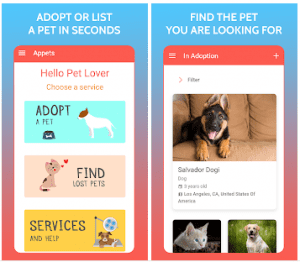The image is a display advertisement likely seen on a website, featuring two side-by-side smartphone screenshots. The background of the entire ad transitions from sky blue at the top to purple on the sides, blending gradually into a soft shade of pink.

The left screenshot showcases a user interface with a red header and a white background. At the top, written in white uppercase letters, is the phrase, "ADOPT OR LIST A PET IN SECONDS." Below, it greets the user with "Hello Pet Lover" and an invitation to "Choose a Service." Three colorful boxes are displayed underneath: the first box is blue and says "Adopt a Pet," the second is pink and reads "Find Lost Pets," and the third is yellow, labeled "Services and Help."

The right screenshot features the heading, "Find the Pet You Are Looking For." It includes a photograph of a dog, likely a German Shepherd or a mixed breed, sitting on a tan-colored sofa. The dog is named Salvador Dogi, a playful twist on words. Description details reveal that Salvador Dogi is two years old and located in Los Angeles, United States. Beneath this main image are two smaller side-by-side photos: one shows the head of a nearly white cat, while the other depicts a light gray dog with very light brown fur around its head.